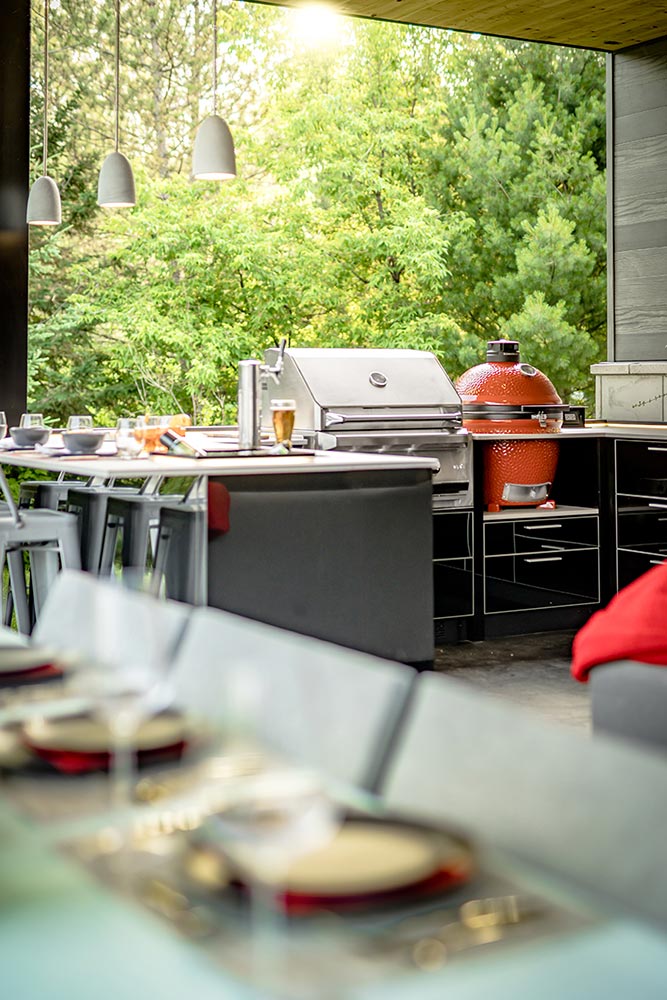This color photograph, vertically oriented, beautifully captures an inviting, modern open-air patio kitchen that seamlessly blends into a sunlit grove of trees in the background. The setting is stylish, with a wooden overhang roof and three elegant pendant lights hanging from white rods above, casting a warm glow. Centered in the image is a stainless steel grill, accompanied by a red-orange, dome-shaped pizza oven with a black cylindrical top and a pressure gauge, both positioned on a sleek, U-shaped metal countertop. Adjacent to these are a beer tap and several yellowish drinks lined up, contributing to the lively atmosphere. The left side features gray stools and a gray counter with multiple bowls and glasses, while the purposefully blurred foreground reveals a formal dining tabletop with metallic red and ceramic plates, possibly gold cutlery, and wine glasses, hinting at a meal ready to be enjoyed. The overall scene exudes a contemporary and welcoming feel, perfectly suited for a stunning outdoor culinary advertisement.